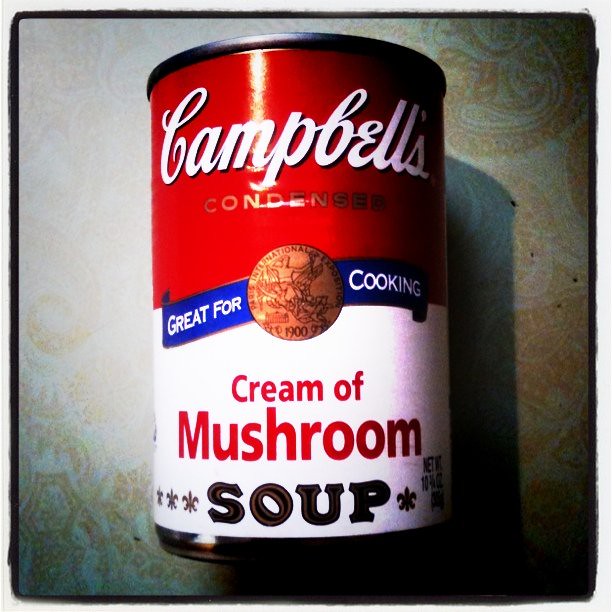A detailed photograph features a Campbell's Cream of Mushroom soup can, prominently positioned lying flat on a richly patterned paisley cloth in striking blue and gold hues. The iconic Campbell's can is showcased with its classic red and white design: "Campbell's" is elegantly scripted in white against the red top half of the label. Just below, the label transitions into white, displaying "Cream of Mushroom" in bold red letters. At the bottom, "Soup" is adorned in stylized black and gold lettering, flanked by delicate fleur-de-lis decorations. A distinctive blue banner runs across the center of the can, announcing "Great for Cooking" — the sole blue accent on the label, harmoniously echoing the blue tones of the background.